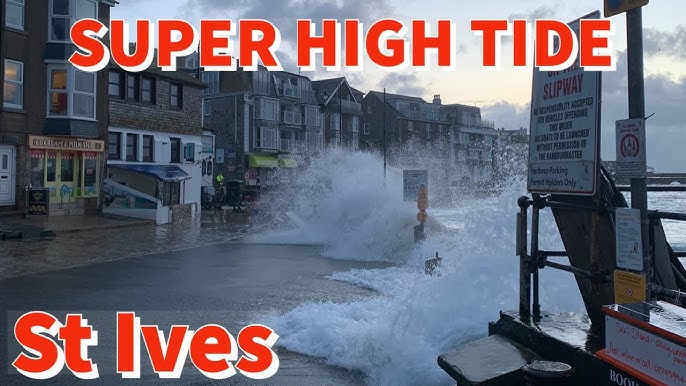The image showcases a dramatic scene of a super high tide event in St. Ives, a picturesque seaside town in the UK. Dominating the image is the bold title in striking red text with an offset white shadow that creates a 3D effect, reading "Super High Tide St. Ives." The scene depicts powerful waves crashing onto the coastal street, encroaching upon the storefronts and houses that line the waterfront. The gray and brown color palette of the town's architecture underscores the intense and somewhat foreboding atmosphere of the event. Among the visual chaos, several signs are visible, including warnings such as "Slipway - No responsibility accepted for vehicles" and "Harbor parking permit holders only," adding to the sense of urgency and alert. The sky above is mostly gray with slight hints of blue, further amplifying the dramatic mood of this high tide scenario.